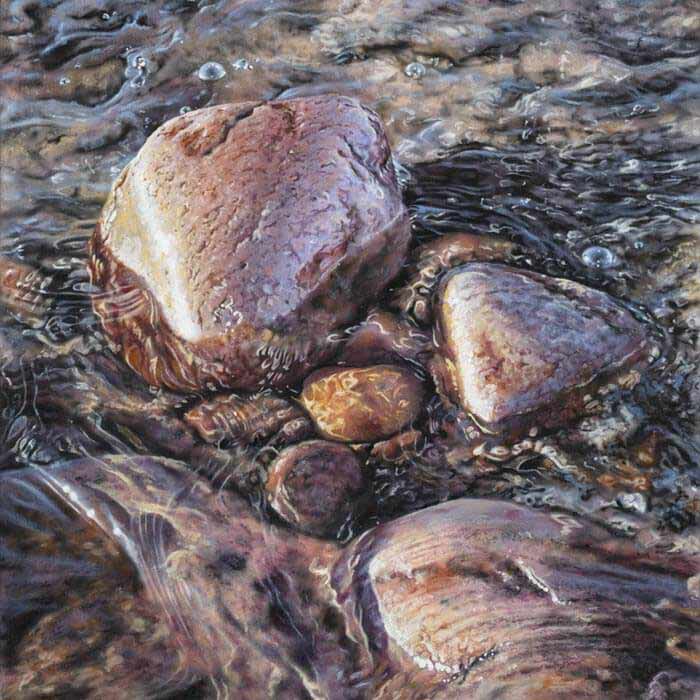The image depicts a close-up, almost macro view of a shallow, flowing stream, where the water is crystal clear, revealing an array of wet, glossy rocks beneath its surface. Dominating the scene, there are two large rocks positioned centrally and another prominent rock in the top left corner. These substantial rocks, characterized by a reddish-brown hue with dark stripes and some black accentuations, display signs of natural wear and divots. Among them, a smaller rock stands out with its vibrant orange color partially submerged in the water. The stream's flow is evident through the ripples, bubbles, and cascading water creating dynamic reflections and curves on the water's surface, giving the appearance of a moment frozen in time. Numerous smaller pebbles and rocks, varying in shades from tan to light red, crowd the riverbed, with some breaking the surface while others lie beneath, all reflecting the sunlight that dances upon the clear, flowing stream.